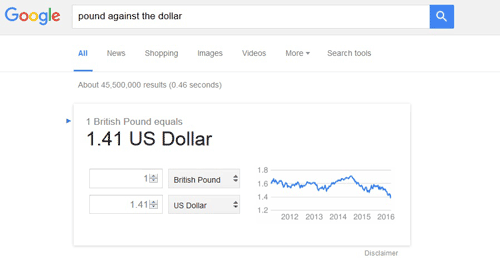The image displays a Google search results page for the query "pound against the dollar." In the upper left corner, the Google logo is prominently featured against a light gray bar that stretches across the top. To the right of the logo is a search bar where the query "pound against the dollar" is entered in black font. Adjacent to the search bar is a blue button with a white magnifying glass icon, representing the search function.

Beneath the search bar is a horizontal menu with options: All, News, Shopping, Images, Videos, More, and Search tools. The "All" category is selected, highlighted in blue with a blue underline indicating its active status.

Below the menu, the search results summary states "About 45,500 results." The primary result displayed shows the current exchange rate: "1 British Pound equals 1.41 US Dollar." An interactive tool is featured just below this, allowing users to adjust the amounts in pounds and dollars to see the equivalent values in real-time.